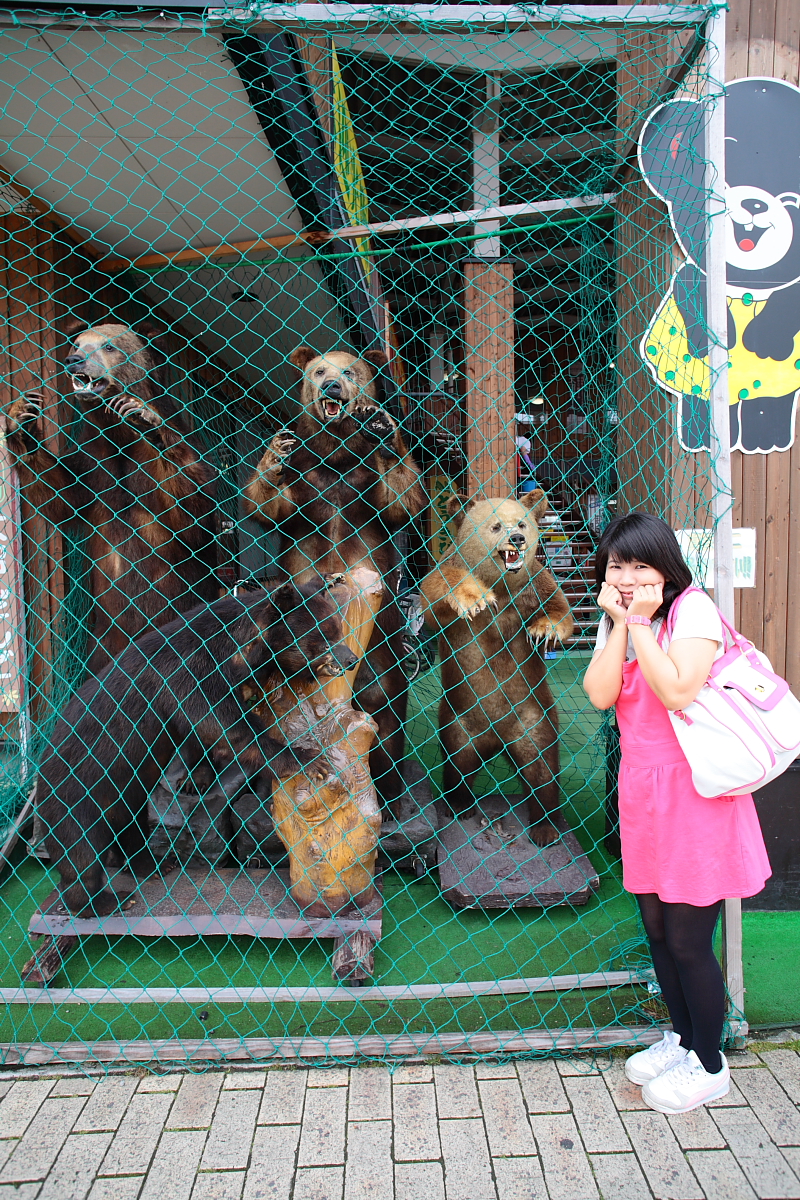This detailed and descriptive caption combines and highlights shared and repeated details from each of the provided captions:

---

In this colorful and delightful image, an Asian woman with shoulder-length black hair and bangs stands in front of a whimsical bear exhibit, assuming an expression of fear with her hands clenched against her cheeks. She is dressed in a bright pink dress with spaghetti straps over a white t-shirt, paired with black leggings and white athletic shoes. Over one shoulder, she carries a large white purse with pink trim matching her outfit. The exhibit behind her features four faux bears within a flimsy-looking netted enclosure with a light framework, resembling more of a playful scene than a serious barrier.

Three of the bears are standing on their hind legs in menacing, rearing poses with open mouths, displayed teeth, and outstretched claws, while the fourth bear, in the foreground, leans forward with its front paws on a tree stump segment. Depicting a family-like setup, the displays might remind one of a mother bear and her cubs. The enclosure’s floor is covered in green astroturf, and each bear stands on stone-grey platforms. Adding to the charm, a cheerful cartoon panda bear dressed in yellow smiles from a sign on the right side. The scene is set on a white brick patio surface, underlining the playful and staged nature of this amusement park attraction, where the woman poses, elegantly accessorized, evoking the blend of humor and a touch of thrill in the captured moment.